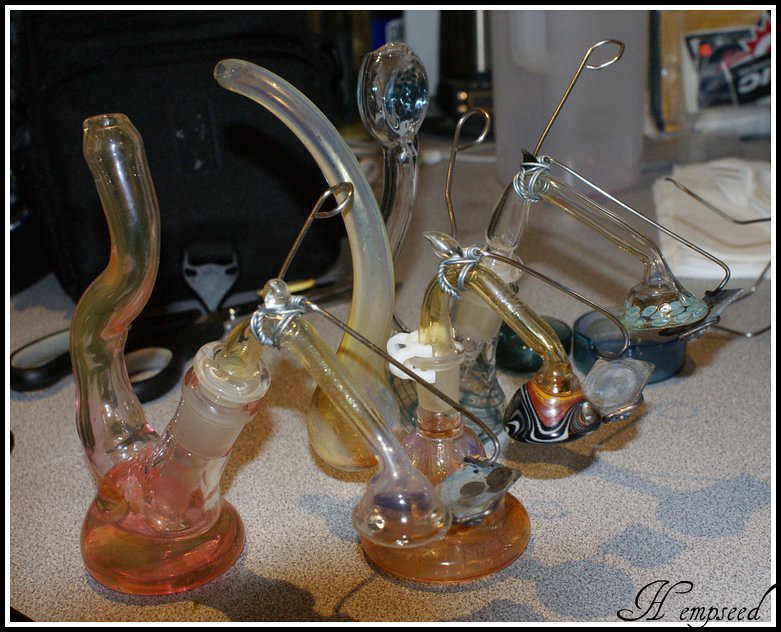This indoor photograph captures a detailed display of six intricately hand-blown glass water pipes, commonly used for smoking marijuana. These elaborate glass pieces, each featuring multiple connected parts, are arranged on a hard surface, possibly a desk or table. The pipes demonstrate a blend of artistry and functionality, with each unit comprising separate round bases and interconnected glass tubes. Some of the tubes arch gracefully, with one end descending into a dome-like structure. Various pipes are wired together, suggesting an intricate assembly, with certain pipes showcasing wires that extend from one part to another.

The glasswork on several pipes is adorned with distinctive designs, including black and white stripes with orange and red accents, enhancing their aesthetic appeal. These pipes have a yellowish tint, indicating signs of use. Additionally, there's visible water in the bases of some of the pipes. A small label that reads "H, hemp seed" can be seen at the bottom, hinting at a branding or a specific theme in the collection. The overall scene suggests a chemistry-like setup tailored for enthusiasts, highlighting both the functional and decorative aspects of these glass artifacts.